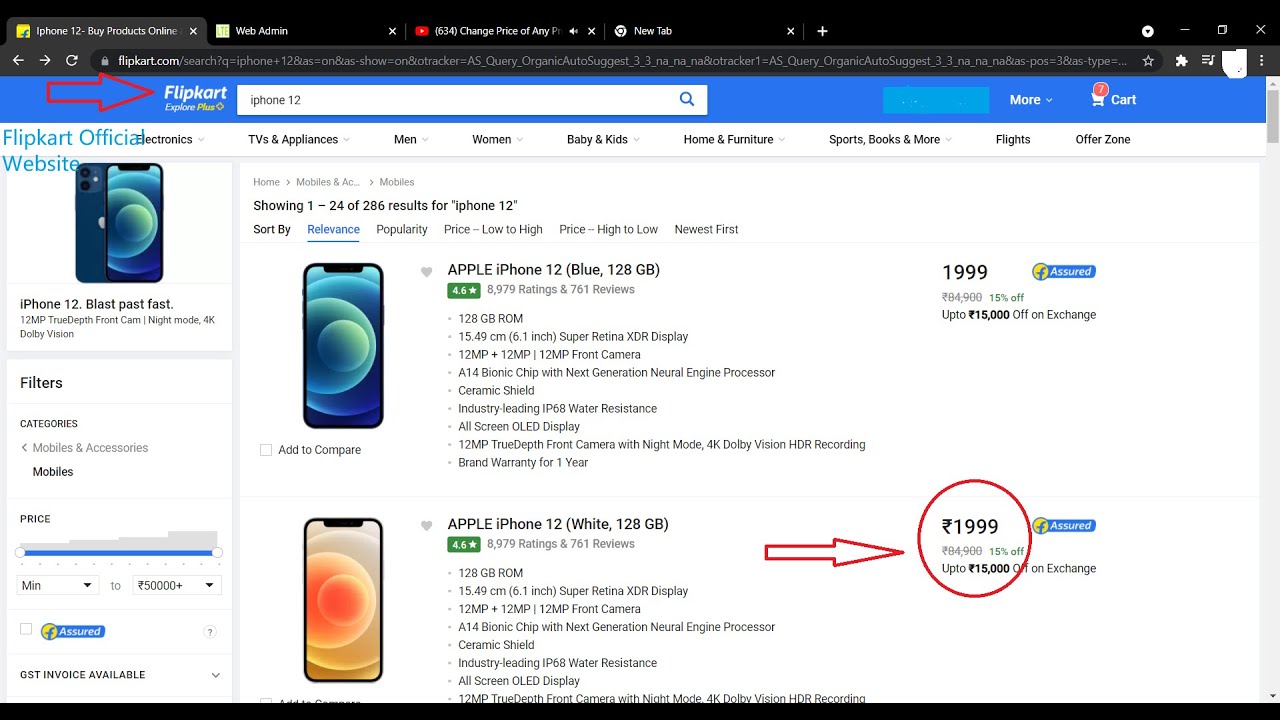This image captures a section of the Flipkart official website, specifically focused on various Apple iPhone 12 models. At the top of the page, prominent headings such as "iPhone 12 byproducts online," "web administration," and "Flipkart Explorer Plus" are displayed. The search engine box displays "iPhone 12," indicating a search for this product. The site navigation bar includes categories such as electronics, TVs and appliances, men's and women's fashion, baby and kids' essentials, home and furniture items, sports books and more, flights, and the offer zone.

The page is showing 1 through 24 of a total of 286 results for iPhone 12 models, currently sorted by relevance with other sorting options available: popularity, price low to high, price high to low, and newest first. The first item listed is the Apple iPhone 12 in Blue with 128GB of storage. This model has received a 4.6-star rating from 8,979 ratings and 761 reviews. Detailed specifications include 12GB ROM, a 15.4 cm (6.1 inch) Super Retina XDR display, dual 12MP rear cameras, a 12MP front camera, an A14 Bionic chip with a next-generation neural engine, ceramic shield, industry-leading IP68 water resistance, and an all-screen OLED display with night mode for the front camera. It also supports 4K Dolby Vision HDR recording and comes with a one-year brand warranty.

The product listing below features the Apple iPhone 12 in White with similar specifications. On the left side of the page, there is a sidebar with a highlighted slogan, "iPhone 12 Blast Pass Fast," and options for filtering categories of mobiles and accessories with price ranges from ₹5 to ₹50,000.